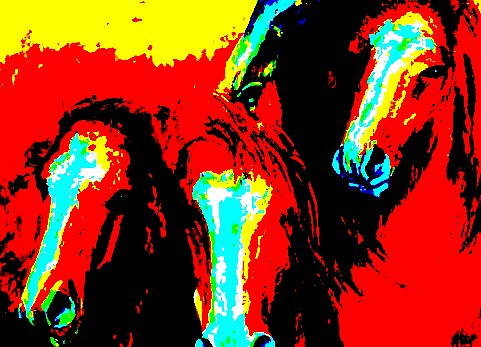The image is a colorfully altered, landscape-format photograph of four horses, focusing prominently on their faces. The photo has been digitally manipulated, creating a vivid, psychedelic color scheme with hues of red, yellow, blue, teal, and black replacing the natural colors of the horses. The manipulation results in a unique negative-like effect.

At the top, the colors transition from bright yellow on the left to black on the right, with intermittent splashes of green and a very light teal color. The horses’ faces, which are mostly outlined in black, feature gradients of color that change from whitish, yellowish, and bluish tones at the top to shades of red and black at the bottom. Each horse has a distinctive white stripe running from its forehead to its nose.

While you can see the majority of the horses' faces, one horse has its nose slightly cut off and another's eyes are not visible. This gives the illusion that the photo was zoomed in a bit too much. The bottom right section displays a vivid teal and dark blue hue, with the faint outline of a signature in black ink, though it’s indistinguishable. Despite the out-of-focus effect and the somewhat chaotic application of the filter, the image intriguingly draws the eye to the abstract representation of the horse heads facing towards the bottom left corner.